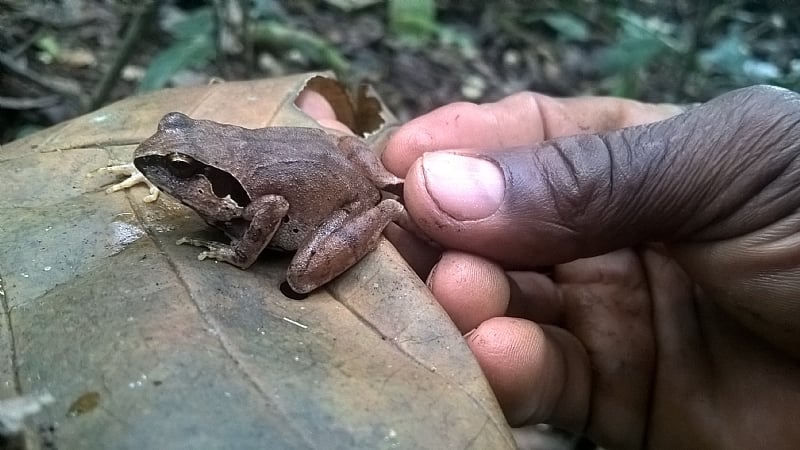In the photograph, a small brown frog with distinctive stripes around its eyes is perched on a large yellowish-green leaf. The frog, about the size of a kiwi fruit, faces left, where a black man's hand gently holds its feet with his thumb and index finger, his palm facing the camera. The background, rendered blurry due to a narrow depth of field, reveals a lush, jungle-like environment with green leaves, bushes, and some soil, contributing to the scene's serene yet vibrant setting. The man's hand appears dirty, suggesting he has been working in the soil before encountering this tiny, seemingly apprehensive amphibian. The entire image, wider than it is tall, encapsulates a moment of gentle interaction within a forest-like habitat.